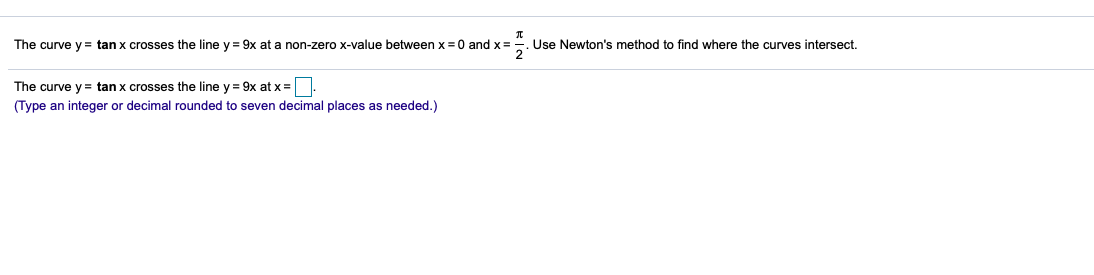A screenshot captures a segment of an unidentified web page, likely associated with mathematics or evaluation. At the top of the screen, there is a thin, horizontal, gray line stretching across the width of the page. Directly below this, a mathematical problem is presented, likely from a subject such as trigonometry or calculus.

The problem reads: "The curve \( y = \tan(x) \) crosses the line \( y = 9x \) at a non-zero \( x \) value between \( x = 0 \) and \( x = \frac{\pi}{2} \). Use Newton’s method to find where the curves intersect."

To reiterate, the text specifies: "The curve \( y = \tan(x) \) crosses the line \( y = 9x \) at a non-zero \( x \) value between \( x = 0 \) and \( x = \frac{\pi}{2} \). Use Newton’s method to find where the curves intersect."

Below this, there is an input prompt: "The curve \( y = \tan(x) \) crosses the line \( y = 9x \) at \( x = \)". Following this sentence is a blue box designated for the user to input the answer.

Further instructions specify: "Type an integer or decimal rounded to seven decimal places as needed."

This concise screenshot ends with no other visible content.